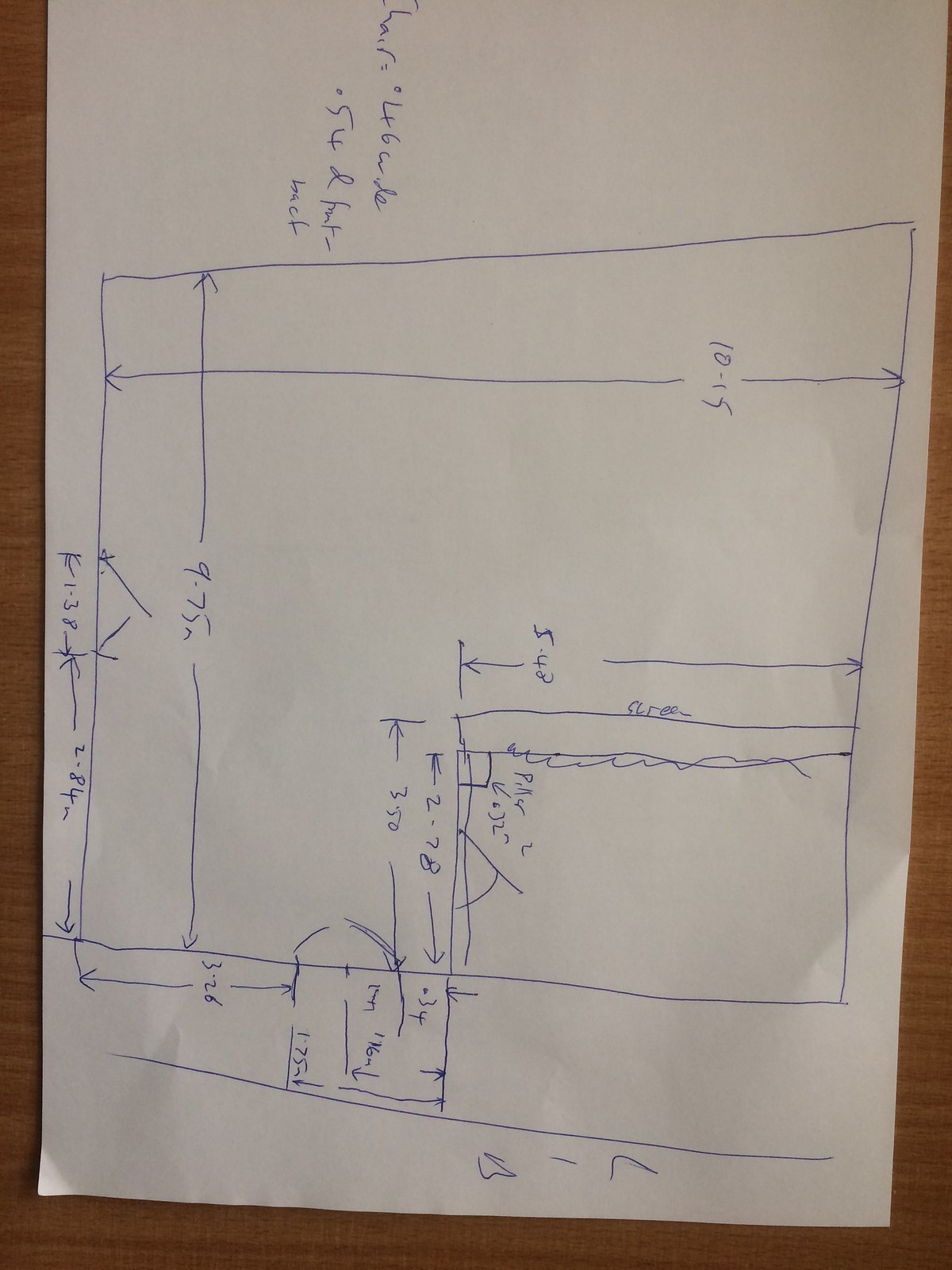This image depicts a handwritten diagram featuring detailed dimensional annotations, likely related to a technical or architectural plan. Along one side, the term "LIB" is prominently noted, which could potentially signify "library" or an acronym pertinent to the context, though its exact meaning is unclear. Centrally located in the diagram is a square-shaped area with an array of arrows. Vertical arrows within this area are marked with "10-15," possibly indicating a measurement range though its exact unit and context are ambiguous. 

A horizontal arrow spans the square with the notation "9.75 M," suggesting a measurement of 9.75 meters. Additionally, several smaller arrows are scattered throughout both inside and outside the square, each accompanied by numerical values. These arrows point in various directions, including vertically and horizontally, and hint at further specific measurements or instructions, though some of the associated text is difficult to discern. Overall, the document appears to be an intricate layout filled with multiple dimensional and directional indicators, the precise interpretations of which remain partially uncertain.